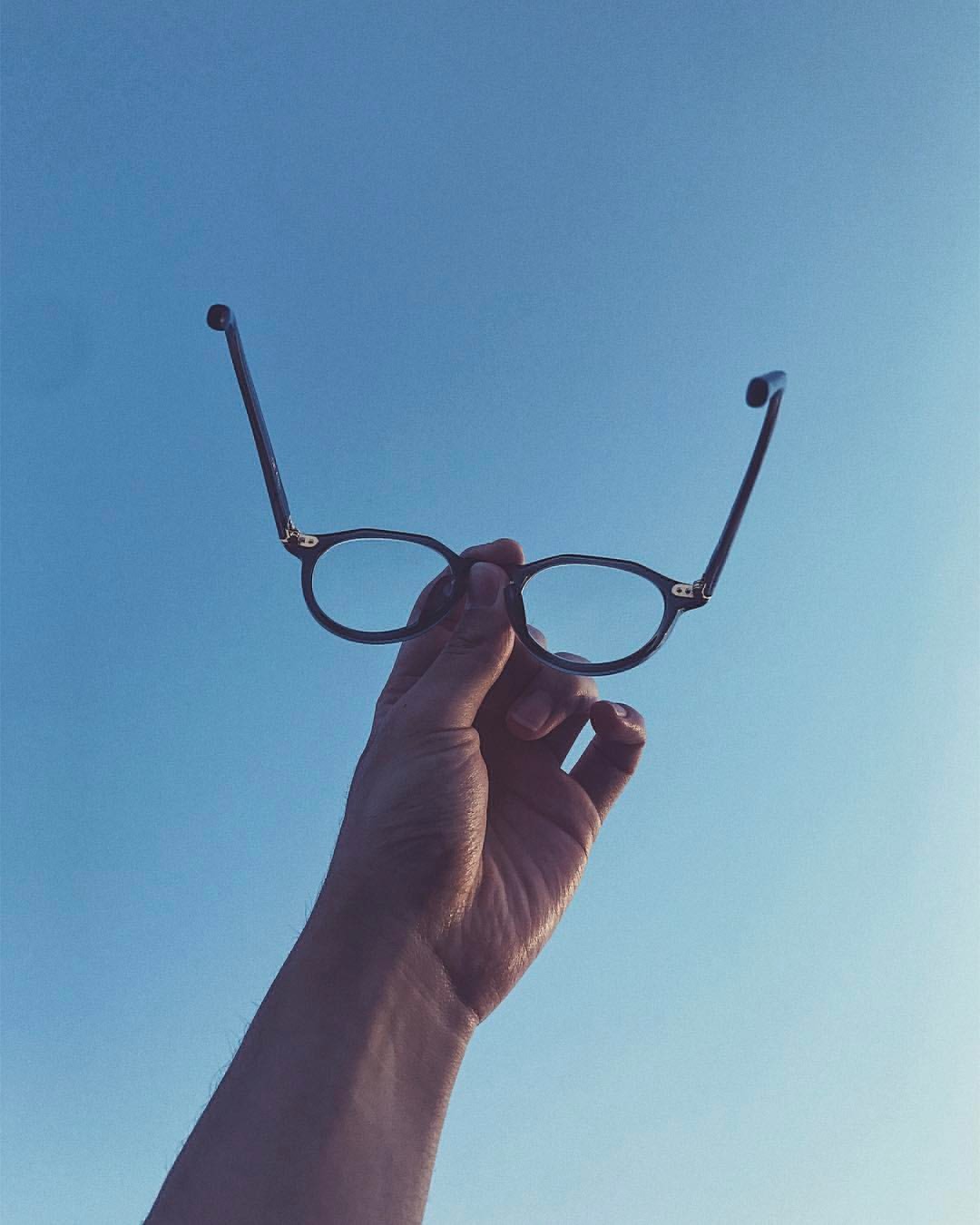The photograph captures a person's left hand holding a pair of eyeglasses up against a clear blue sky, with the hand positioned in the lower left corner of the image. The sky transitions from a lighter blue in the lower right to a darker blue in the upper left, with minimal clouds. The person, likely of Caucasian descent with short, unpolished fingernails, is pinching the bridge of the glasses between their thumb and forefinger while their middle and ring fingers are curled inward, and their slightly raised pinky. The glasses, featuring circular rims and black frames with pronounced silver metal connectors, resemble regular vision eyewear rather than sunglasses. The clear lenses suggest a mild prescription, evidenced by the lack of significant refraction. The photograph seems to depict the moment just after the glasses were taken off, highlighting the reflective light of what appears to be a rising sun.